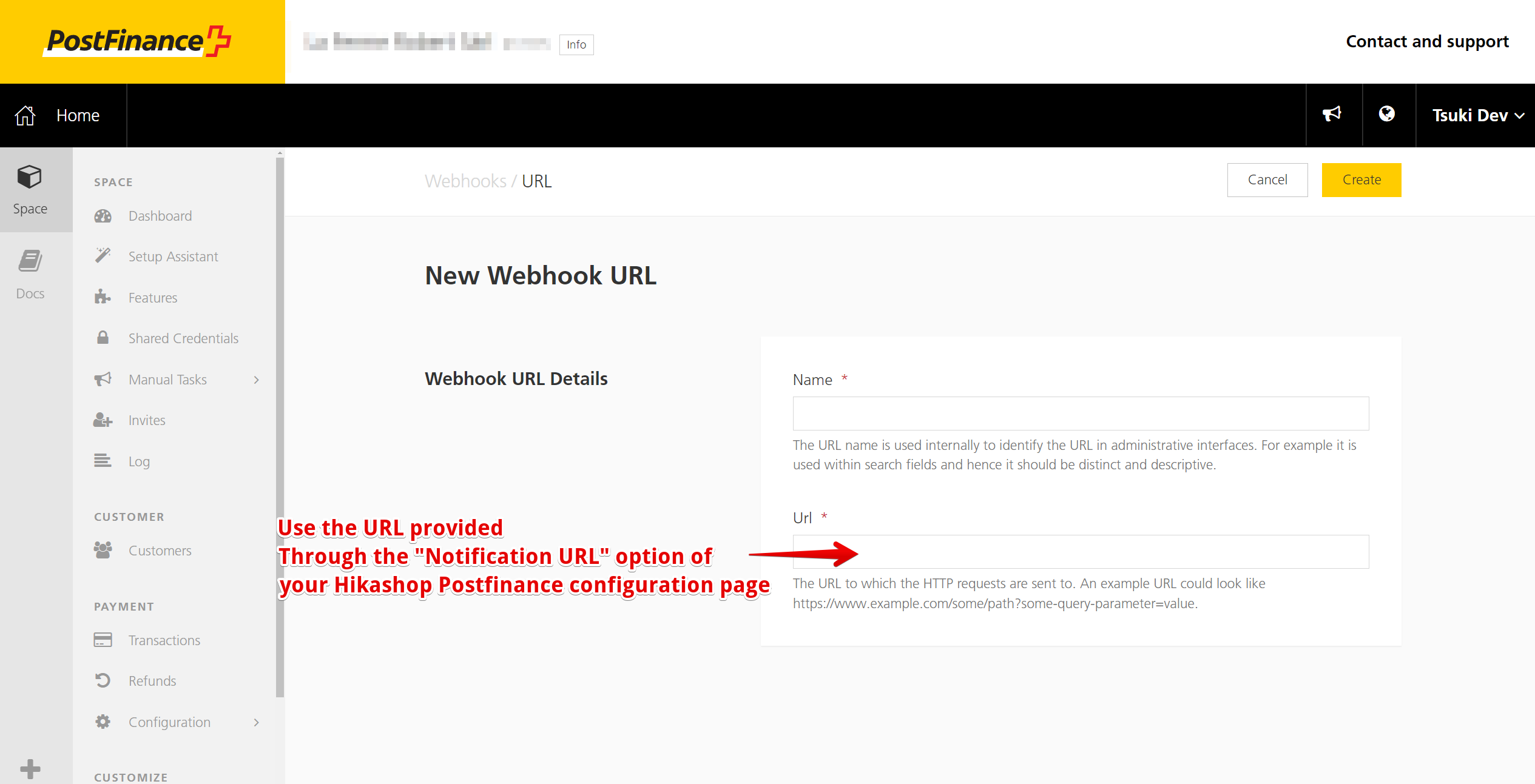This image depicts a post-finance setup interface with a detailed dashboard and multiple options. 

The background of the interface is gold, with text elements prominently displayed. In the top section, there is a clearly marked "Post-Finance" label in white underlined text accompanied by a red plus arrow, indicating the option to add or expand features. To the right of this section, personal information is pixelated for privacy. On the far right, there are accessible options labeled "Contact and Support."

On the left side of the interface is a vertical menu featuring various sections, each accompanied by small icons. The sections include:
- Dashboard
- Setup Assistant
- Features
- Shared Credentials
- Manual Tasks
- Invites
- Log
- Customers
- Payments (with sub-options: Transactions, Returns, Configurations, and a plus icon)
- Configure (or Customize Area)

In the main field of the interface, an administrative task is being set up. The section title reads "New Webhook URL." Within this field, there are placeholders for text and various options, including "Name" and "URL," with a description stating that the URL name is used internally to identify the URL within the administrative interfaces.

However, this field has notably small text, making it challenging to read. A handwritten note in red highlights the URL field, advising users to "use the URL provided through the notification URL option of your HECA shop post-finance configuration page," indicating a level of frustration with the setup instructions.

Overall, the image represents a complex administrative interface with a focus on setting up webhook URLs, providing a mixture of detailed options and some user interface challenges.